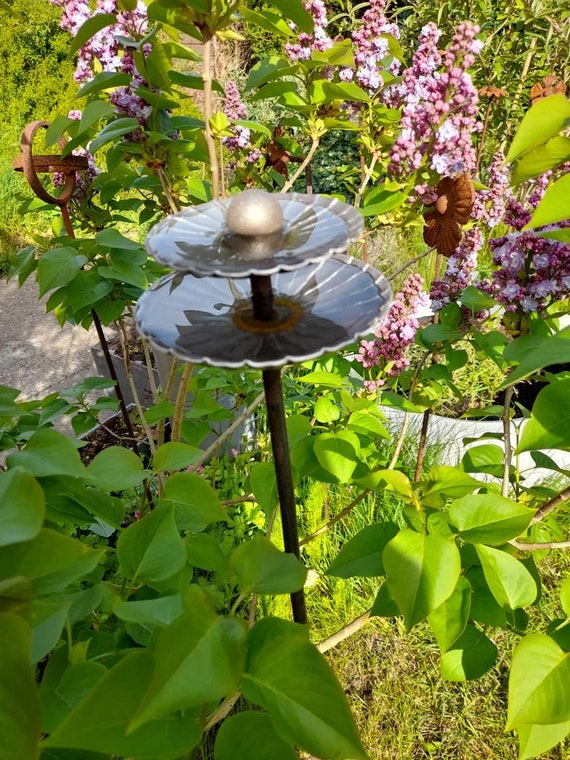The image is a vibrant outdoor scene taken on a clear, sunny day. At the center is a birdbath with two levels; both the base and inner ring are black, while the inner ring features a red accent. Atop the second level sits a polished, white metallic ball. The birdbath, made of rusting metal, has some polished metallic discs resembling shells, possibly functional or decorative. Surrounding the birdbath is a lush garden with an abundance of green leaves and various flowers. To the right are purple flowers, and above them is an open red flower with a yellow center. Further up are clusters of pink and white flowers with bright green leaves. To the left, there is a weathered wooden circle with a spinning element, set against more greenery. In the foreground, there are large green leaves, and the garden floor is a mix of grass, rocks, and dirt. The backdrop includes additional decorations, such as a rusty circular ring and possibly another aged flower ornament, with hints of a concrete path peering through the foliage. The scene captures the intricate details and colors of a well-tended garden bathed in sunlight.